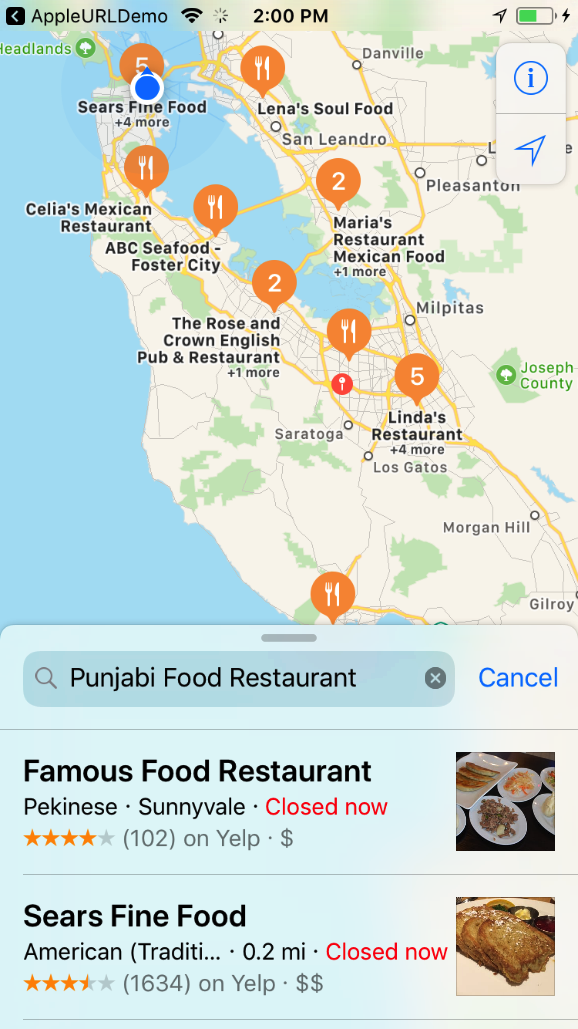The image appears to depict an Apple Maps interface labeled "Apple URL Demo" at the top, indicating that this is a demo version not currently available to the public. The upper section of the display includes a Wi-Fi signal icon, a buffering symbol, a timestamp reading "2 PM," and a battery life indicator that is halfway filled in green.

Central to the display is a map populated with various restaurants, each marked by an orange pin accompanied by a fork and knife symbol, signifying food establishments. One of these pins highlights "Lena's Soul Food," showing its exact location on the map. Below the map area, there is a listing, currently focused on "Punjabi Food Restaurant," with the option to click an 'X' to remove it and perform a new search for other restaurants.

Further down, two restaurant listings are detailed. The first is "Famous Food Restaurant," which offers Pekingese cuisine located in Sunnyvale. The status indicates it is "Closed Now" in red text. This restaurant has a 4 out of 5-star rating based on 102 reviews and includes a small image preview of the dishes available. The second listing is for "Sears Fine Food," which serves American cuisine. It boasts a higher rating of 4.5 out of 5 stars. The price range is indicated by dollar signs, suggesting that the restaurant may be more expensive. Each listing is also accompanied by a thumbnail image showcasing some of the food items offered.